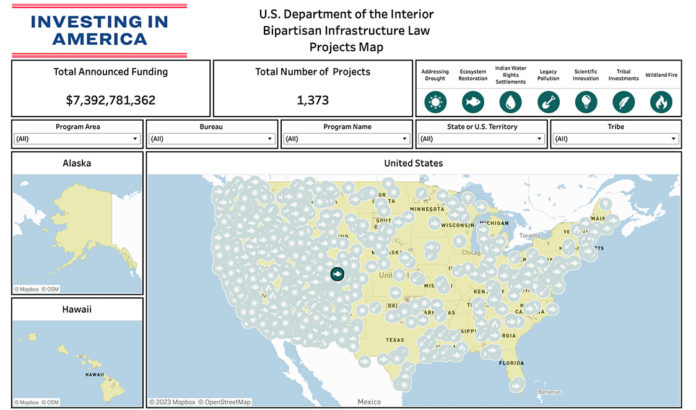The image features a banner at the top reading "U.S. Department of the Interior Bipartisan Infrastructure." Prominently displayed on the left side is the phrase "Invest in America" followed by a list of states involved in the initiative, including Alaska, Texas, Wisconsin, Minnesota, Michigan, and Florida. The total announced funding for the project is an impressive $7,392,781,362, highlighting a significant investment aimed at improving infrastructure across these states.